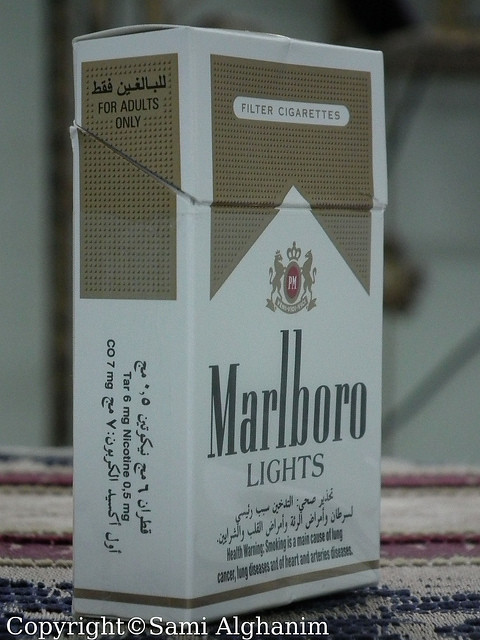The image is a close-up of a pack of Marlboro Lights cigarettes placed on a textured surface that resembles a fibrous material with red, yellow, and purple colors, possibly carpet-like. The pack is positioned at an angle showing both the front and the left side. At the top of the front side, there is a white circle that says "Filter Cigarettes" in light brown lettering, above a light brown background that extends halfway down, forming a V-cut in the center. The Marlboro logo is prominently displayed with two lions facing each other and a crown in the middle, alongside a red circle featuring a white "PM." Below this, "Marlboro" is written in black text, followed by "lights." Further down are three lines of text; one in a foreign language, and below that, a health warning in English: "Smoking is a main cause of lung cancer, lung disease, and of heart and artery diseases."

The left side of the pack features a brown patch with black dots and contains more text. At the top of the patch, another line of foreign characters followed by "for adults only." Towards the bottom, vertical text lists tar and nicotine amounts—"tar 6mg, nicotine 0.5mg"—and "CO 7mg" with additional foreign text. Also on this side is a note of copyright, indicated by a "C" with a circle around it, attributed to Sami Al-Gahimin. The background behind the pack is blurry and out of focus, drawing attention to the cigarette pack itself.